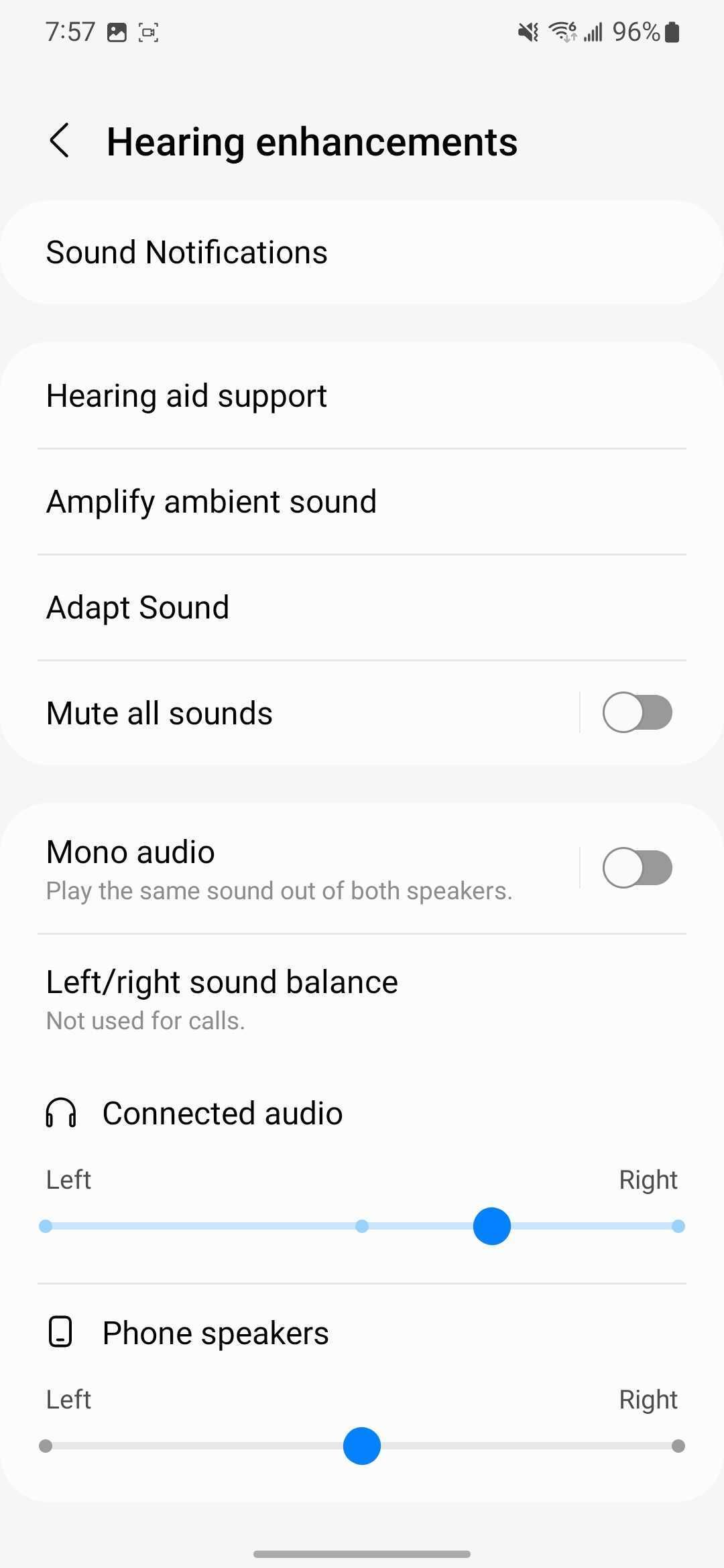The screenshot displays the settings page of a smartphone. At the very top left corner, the time is shown as 7:57, while the top right corner indicates a battery life of 96% alongside other status icons. Directly below this, there is a header featuring a less than symbol (`<`) and the text "Hearing enhancements".

Beneath this header, there is a large white box labeled "Sound notifications". Following this box, a section of light gray color precedes another white box labeled "Hearing aid support". Below this, a light gray line extends horizontally across the screen.

Subsequently, the settings continue with black text options: "Amplify ambient sound" is listed first, followed by "Adapt sound". Further down, there's another gray line marking the "Mute all sounds" option, which is equipped with a toggle bar to switch it on or off.

The final option displayed is "Mono audio, play the same sound out of both speakers," accompanied by yet another toggle bar on the right, allowing users to enable or disable this feature.